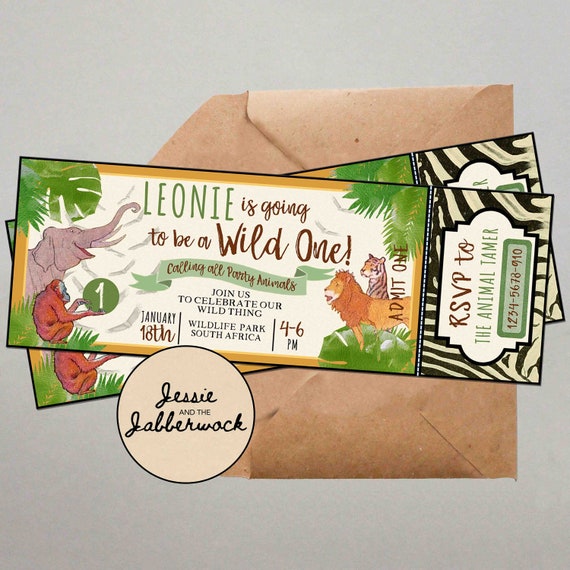The image features a pair of overlapping safari-themed tickets on top of an open brown envelope. The tickets prominently display illustrations of jungle animals, including an elephant, monkey, lion, and tiger. The monkey is holding the number one. The tickets read "Leonie is going to be a wild one" and "Calling all party animals, join us to celebrate our wild thing." The event is scheduled for January 18th from 4 to 6 p.m. at the Wildlife Park in South Africa. An RSVP is requested to the 'animal tamer' at the number 1-2-3-4-5-6-7-8-9-10. Below the tickets, there's a circular emblem that reads "Jesse and the Jabberwock." The overall presentation hints at an invitation for a children's birthday party.